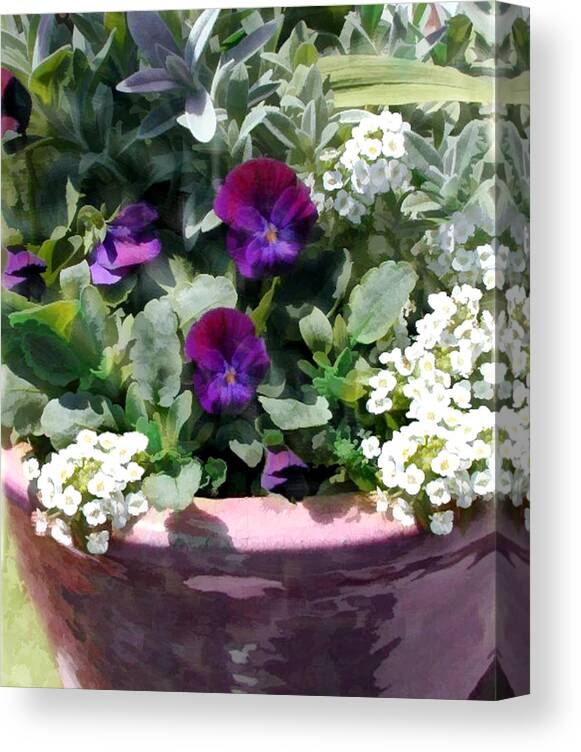This is an image of a painting on a thick canvas, angled slightly to reveal its edges, which are also painted. The painting depicts a vibrant flower pot filled with various flowers and foliage. The pot itself is a very light purple color with visible shadows cast upon it, hinting at bright sunlight. The flowers in the pot are diverse: white miniature blossoms with yellow centers, rich purple flowers that appear to be petunias, and varied shades of green leaves ranging from thick and dark to lighter and more delicate. The intense illumination suggests an outdoor setting, bolstered by the dull green area at the lower left that looks like grass, reinforcing the impression that the scene is set in a sunny garden or lawn.